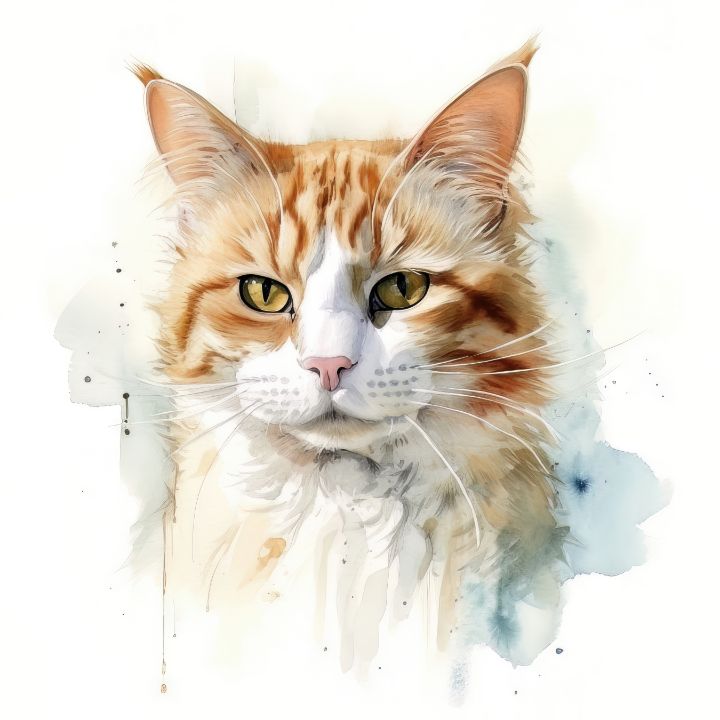The image showcases a beautifully detailed watercolor painting of a tabby cat set against a white background. The cat, positioned prominently in the middle, has a luscious coat of orange and white fur with distinctive dark orange stripes. The fur appears very fluffy, with pointed ears adorned by fur tufts at their tips. The face and ears exhibit intricate detailing, highlighting the cream-colored fur with peachy undertones and some orange hair sticking up.

The cat's eyes are a striking combination of yellow and black, with a shiny appearance that captures its intense gaze directed at the viewer. The nose area is white, leading to a pink nose, and the long white whiskers stand out prominently. Around the edges of the painting, light blue and teal watercolor textures fade into the white background, adding a subtle yet elegant border that slightly blends with the cat’s fur, almost giving a shadowed effect. The overall effect is a lifelike portrayal of an adult tabby cat, radiating softness and cuteness.